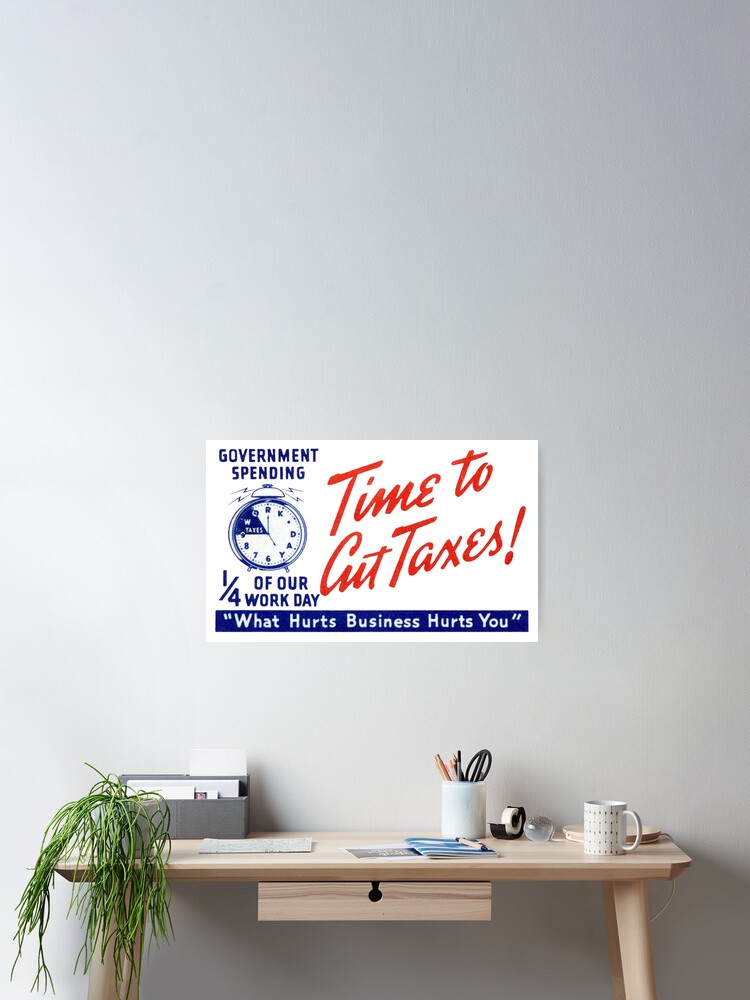This photograph captures a well-organized home office set against a light gray or off-white wall. The focal point is a modern pine wood desk situated towards the bottom right of the image. The light brown desk, featuring a single drawer with a distinctive keyhole-shaped pull, supports an array of office essentials: a small, overgrown green plant drapes down its side, a gray letter holder for mail and paperwork, and a variety of stationery items including a pencil holder filled with pencils, pens, and scissors. Additionally, the desk holds a cream-colored coffee cup with a matching handle, a tape dispenser, some papers and pamphlets, and a flexible, clamp-on desk lamp positioned to the right.

Mounted above the desk is a small, visually striking poster with a white background and red script reading "Time to Cut Taxes." The poster also includes additional elements like the phrases "Government Spending" in blue text, a graphic of an alarm clock, and "One-Fourth of Our Workday." At the bottom of the poster, in a blue rectangular banner with white text, it reads "What Hurts Business Hurts You." This detailed arrangement not only highlights the desk's functionality but also adds a touch of personal and political expression to the workspace.